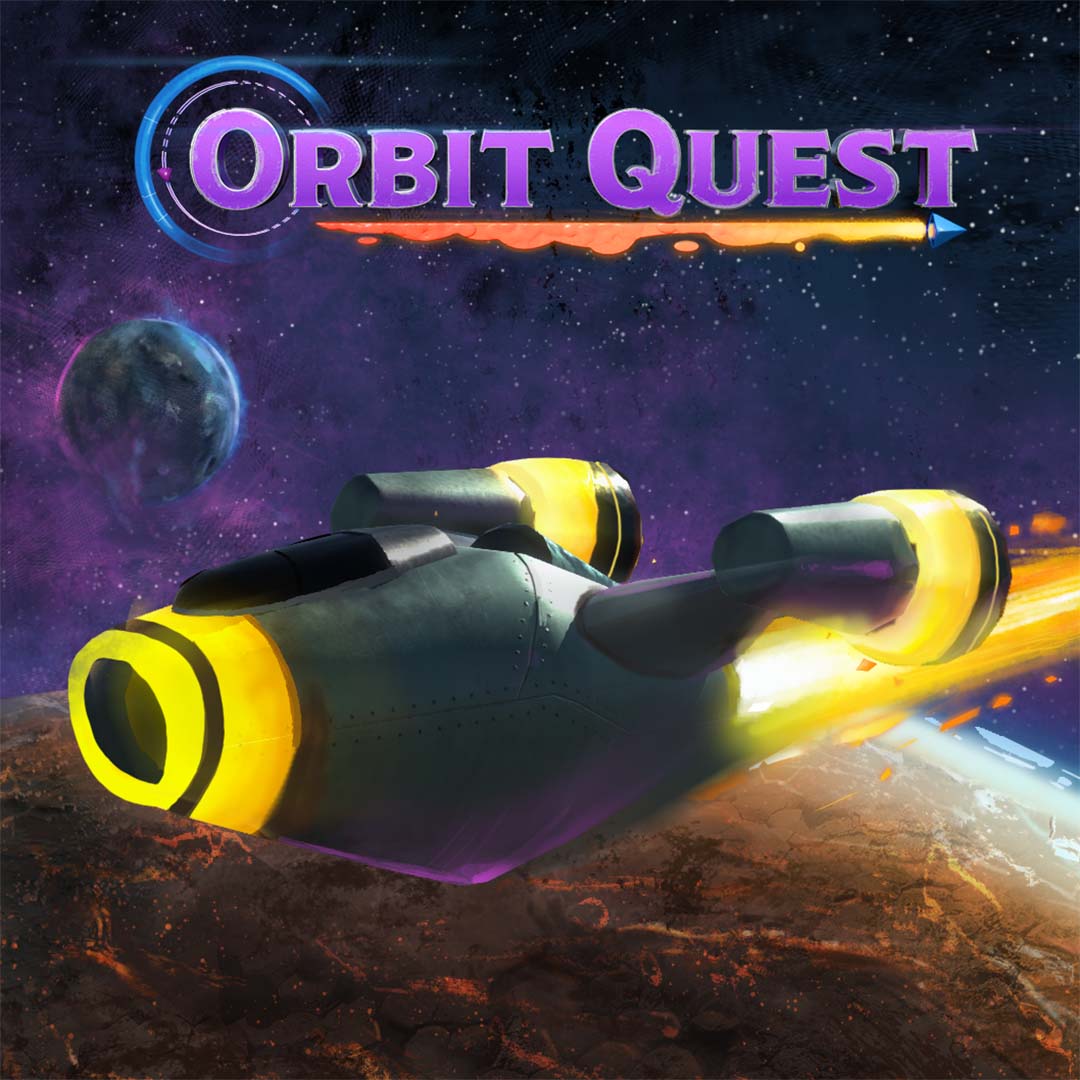The image is a promotional poster for a video game or movie titled "Orbit Quest." The title "Orbit Quest" is prominently displayed at the top in large, bold, purple letters with a thin light gray outline and a 3D effect. The letter "O" in "Orbit" is stylized with an orbital pattern consisting of dashed gray lines, a smaller red dot, a larger blue circle, and possibly a white smaller ring, all set against a starry backdrop that transitions into a purple nebula.

Below this title, there is an underlining that transforms into an arrow, with a blue tip and flames forming the underline. Dominating the foreground is a large, black and yellow spaceship with horizontal symmetry. The spaceship features yellow thrusters at the rear that emit bright flames, and the nose of the ship is painted yellow. The ship has two conical protrusions at the back.

The background of the image is an expansive outer space setting starting with a black gradient that transitions into purple clouds or haze. Midway down on the left side, there's a planet with various shades of blue, suggesting an earthly or water-like appearance. At the bottom of the image, filling the entire lower portion, is another planet, predominantly brown with red lines suggesting fiery activity or movement.

The entire composition captures a dynamic scene of space exploration and adventure, perfectly encapsulating the essence of "Orbit Quest."